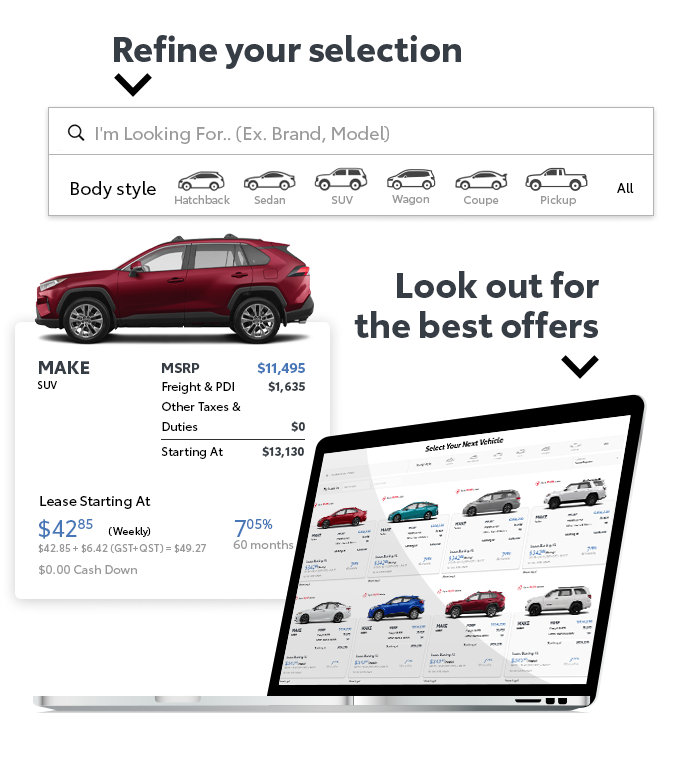In the image, you see a user interface designed for car selection. At the top, there is a black header with the text "Refine Your Selection" and a downward arrow next to it. Below, a white search bar features a black magnifying glass icon. Inside the search bar, gray placeholder text reads "I'm looking for... (e.g., brand, model)". 

Under the search bar, there's a separator line followed by the heading "Body Style" in black text. Beneath this heading, various car types are listed with corresponding images: Hatchback, Sedans, SUV, Wagon, Coupe, Pickups, and an option labeled "All" in black.

Prominently displayed below the body style options, there is an image of a red SUV. Pertinent details about this vehicle are provided: "Make: SUV, MSRP: $11,495, Freight and PDI: $1,635, Other Taxes and Duties: $0. Starting at $13,130. Leasing starts at $42.85 weekly plus $6.42 GST and QST, amounting to $49.27 with $0 cash down, at a 7.05% interest rate for 60 months."

Further down, there's a prompt: "Look out for the best offers" accompanied by a downward arrow. Finally, the image features a tablet displaying two rows, each with four different car images under the header "Select Your Next Vehicle."